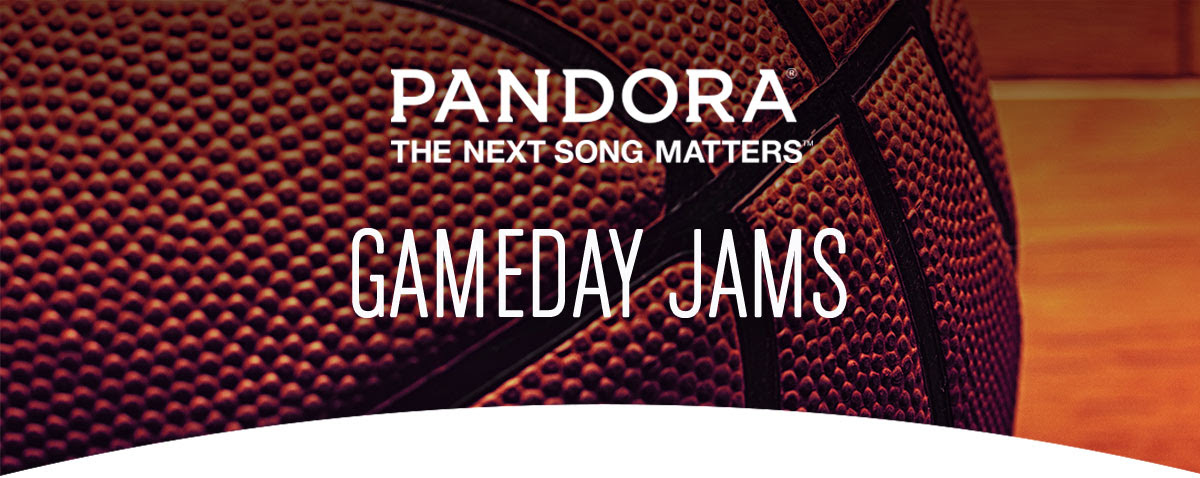The image appears to be a vibrant advertisement graphic featuring the familiar Pandora logo at the top with the tagline, "The Next Song Matters," in slightly smaller white text. Below this, "Game Day Jams" is prominently displayed in a larger white font, distinct from the Pandora typeface. The background showcases a close-up of an orange leather basketball, its textured surface and black lines emphasizing its realism. This basketball occupies about two-thirds of the image, positioned primarily on the left side. A subtle portion of a wooden basketball court is visible on the right, suggesting the setting. The overall shape of the image is unconventional, with a noticeable white, curved bulge at the bottom, breaking the rectangular form.